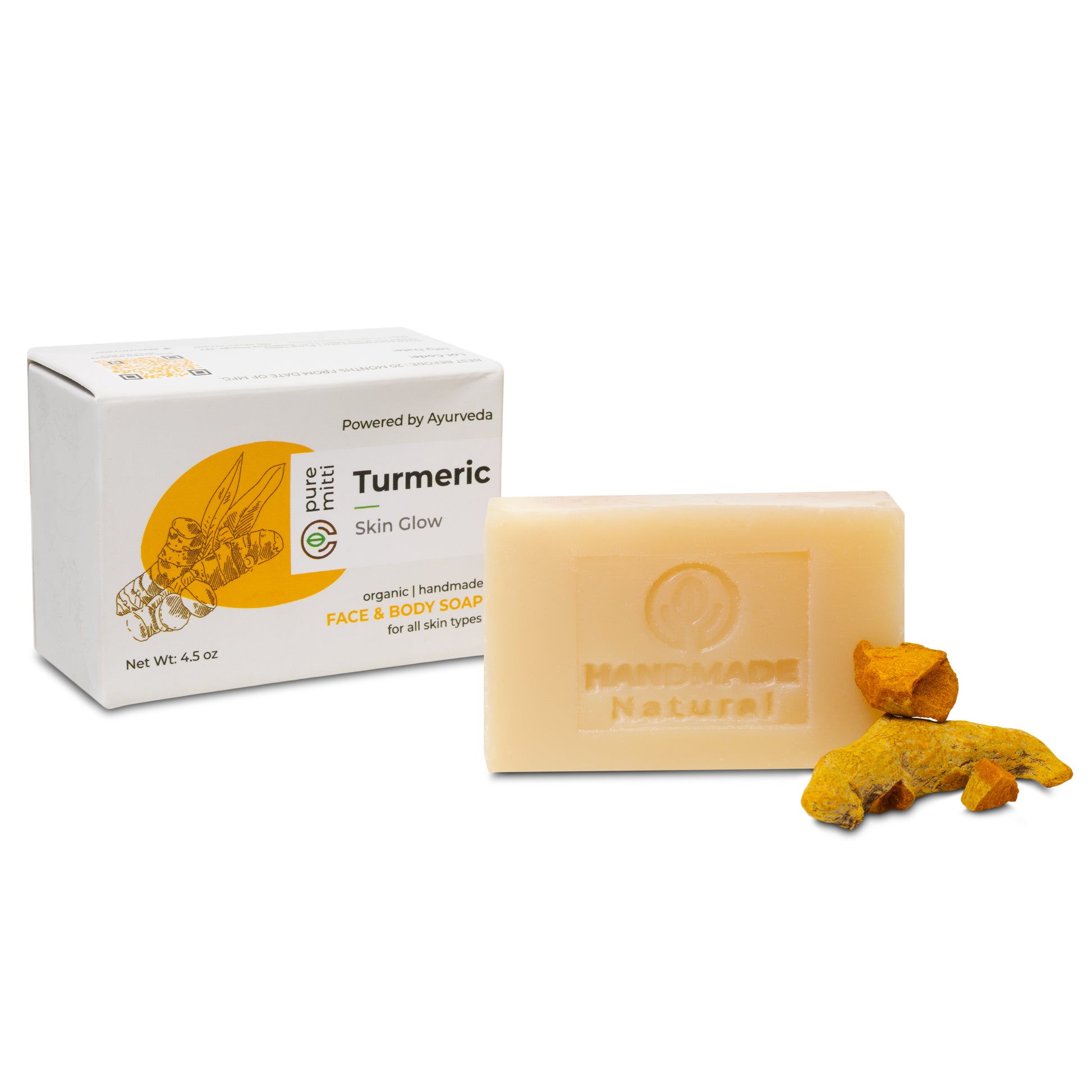The image is a color photograph designed for advertising soap, set against a solid white background. On the right-hand side, there is a translucent, creamy, vanilla-white bar of soap with an imprint that reads "Handmade Natural" accompanied by a leaf logo inside a circle. This soap is slightly peach or beige in color. Adjacent to the soap on its right side, there are several yellow spice objects, likely turmeric chunks. To the left of the soap, the box it came in is displayed at a slight angle. The white cardboard packaging is detailed with text, starting at the top: "Powered by Ayurveda" followed by "Turmeric" in bold black letters, and "Skin Glow." A vertical inscription reads "Pure Meaty," and there is an orange circular logo with a turmeric image next to it. Below, it states, "Organic" with a vertical slash through "Handmade" in orange letters, and then "Face and Body Soap," "For All Skin Types" in black letters. At the bottom left corner, it indicates "Net Weight 4.5 oz" (or 4.5 ounces). The left side of the packaging also features an image of turmeric, reinforcing the natural ingredient theme.